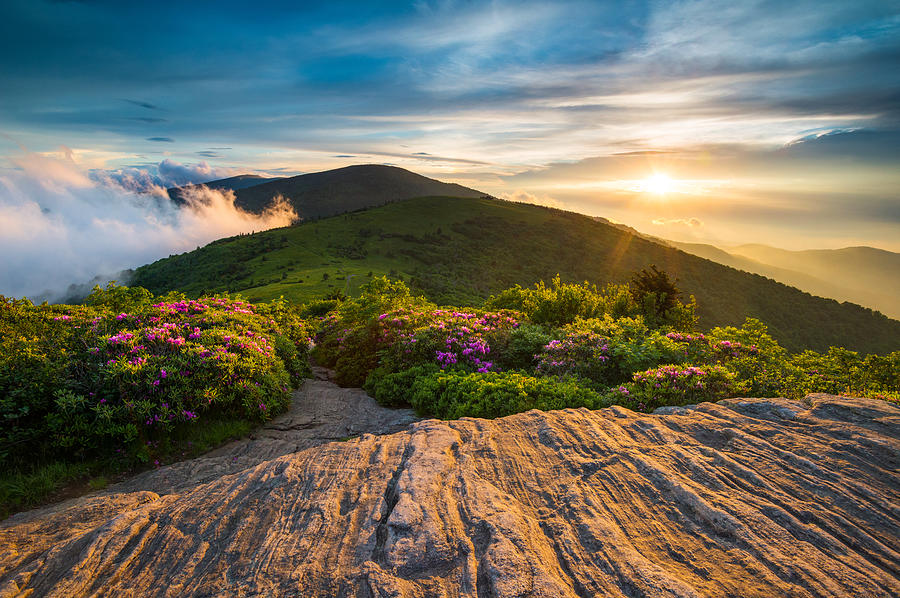The image captures a breathtaking scene from a high vantage point on a green, mountainous terrain. As the sun sets on the right, it bathes the area in dramatic light, casting vivid hues across the landscape. The sky is a hazy blue, dotted with soft, fluffy clouds that stretch from the foreground up into the distance, almost resembling smoke. The lush greenery is interspersed with striking, colorful flowers, predominantly pink and purple, resembling tulips. The foreground showcases a rocky, barren patch of earth, contrasting with the lush surroundings. Farther away, rolling hills and additional mountains create a layered, ethereal vista reminiscent of New Zealand or a fantastical landscape from Lord of the Rings. The scene is devoid of people, making it feel serene and untouched, perfect for capturing moments like wedding or engagement photos.